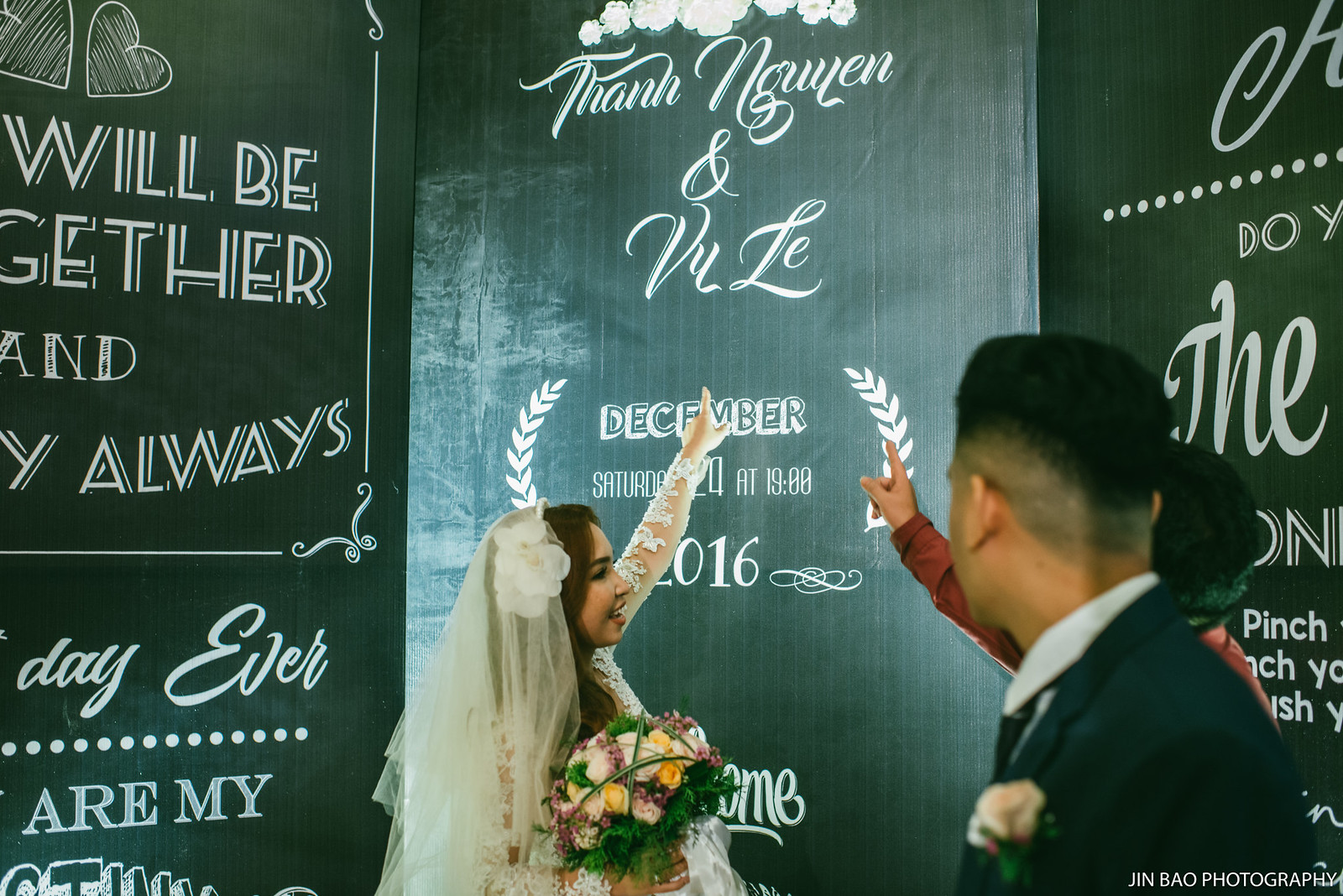In the image, we see a central scene featuring a bride and groom, suggesting a wedding setting, which could be either indoors or outdoors. The background prominently displays a tan poster with heart graphics on the top left, containing text that reads, "We'll be together always," followed by "Than Win" and "Vu-Le," along with the date "December, Saturday 24th, 2016, at 19:00."

In the forefront, a man and a woman, presumably the groom and bride, are the main focal points. The groom, positioned slightly to the left, has black hair and is dressed in a black suit with a white shirt. Next to him is the bride, wearing a white dress and a headscarf, holding a bouquet of flowers. She is pointing towards the names on the poster. A third individual, standing directly behind the groom, wears a maroon suit and is also pointing at the names on the poster.

The image contains a variety of colors such as green, white, purple, yellow, brown, tan, and black, adding to its vividness and depth. Black signs are placed around the couple—one on the left and one on the right—though these signs are partially cut off and unreadable. This detailed scene encapsulates the joyous moment of an Asian bride and her groom on their wedding day amidst celebratory decor and significant signage.